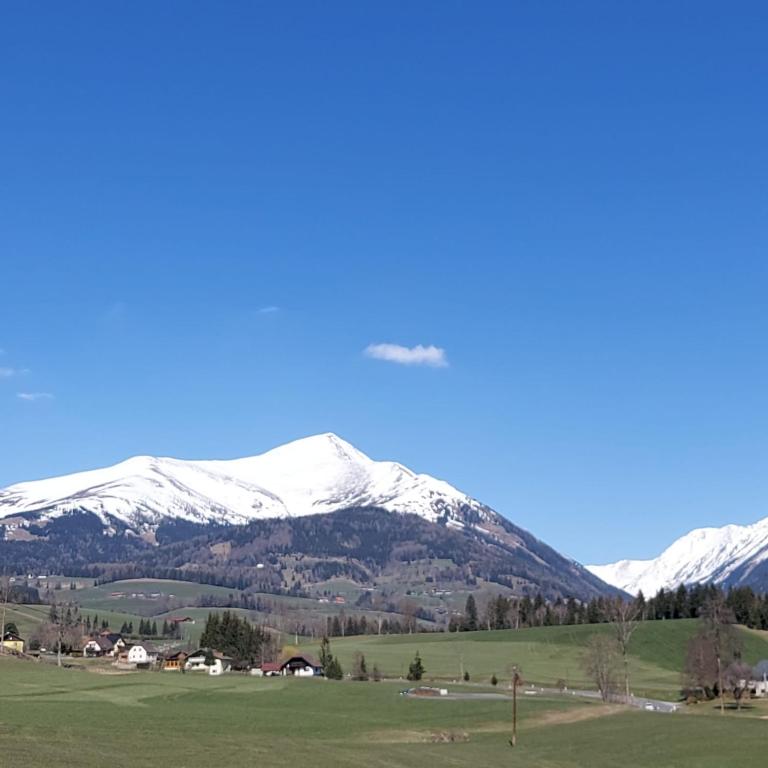This captivating image showcases a serene mountain landscape, characterized by rolling green hills dotted with houses and trees. The freshly mowed grass enhances the lush greenery that envelops the scenery. A road, visible with a few cars, winds through a cluster of homes nestled closely together amidst the abundant foliage. As the terrain ascends, the houses become sparse, giving way to the rugged foothills and further up, the mountaintops are adorned with pristine white snow. The snowy peaks, juxtaposed with the lush lower elevations, create a striking contrast. The sky above is a clear, vibrant blue, punctuated by a few wispy clouds, with one prominently centered in the image and a few more on the left. This beautifully composed image captures the sublime beauty of nature's diverse elements, from verdant pastures to majestic, snow-capped peaks.